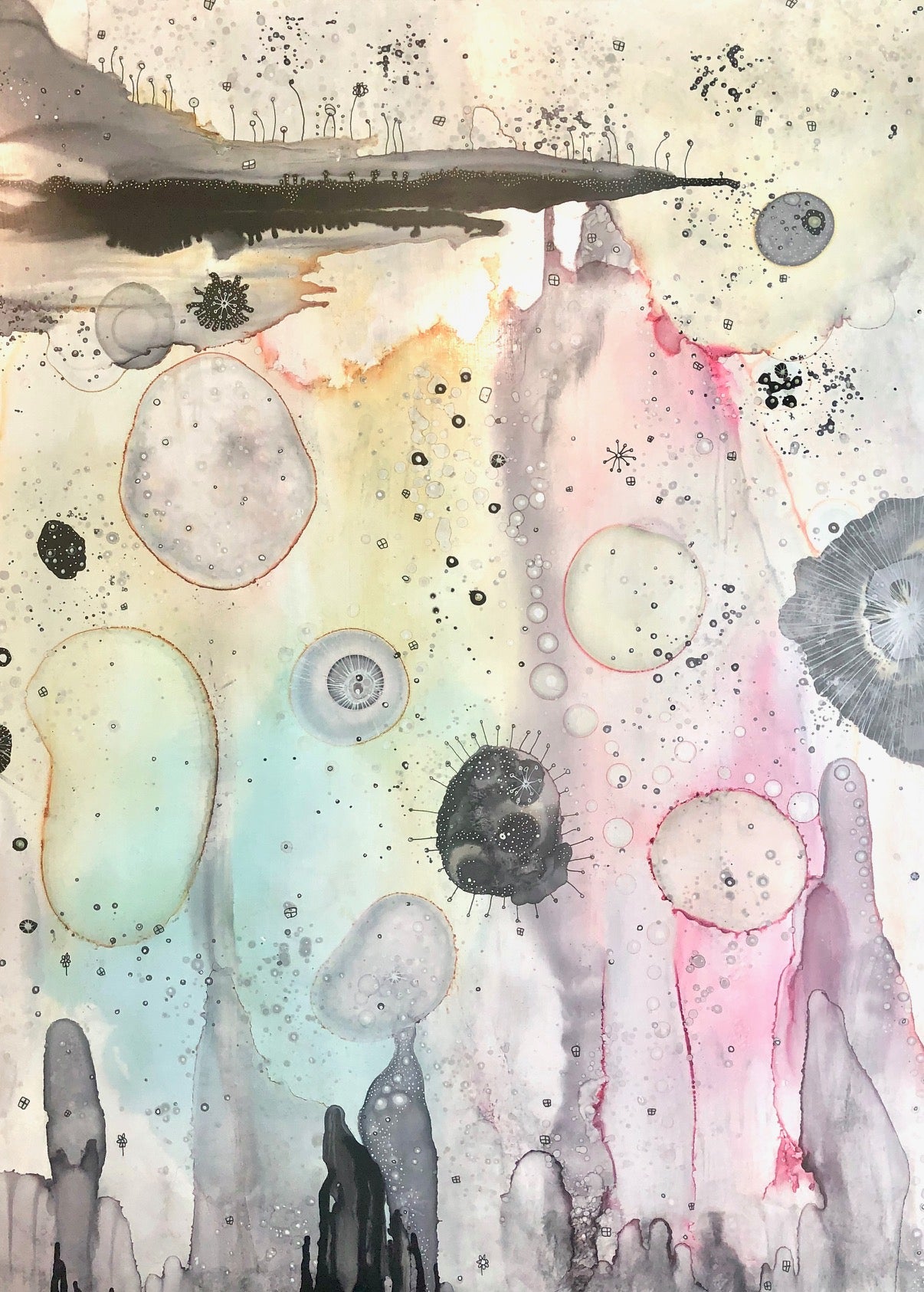This vertical canvas of abstract art features a chaotic yet intriguing mix of forms and hues. Predominantly characterized by muted colors, the base is a blend of whitish or beige tones, punctuated by dynamic elements of primarily gray, light pastel blue, and faint yellow. A bold black stroke stands out in the top left corner, accentuating the piece's dramatic flair.

The painting is composed of various shapes, including circles, ovals, and egg shapes, intermixed with lines and dots. Some of these orbs and bubbles, tinted in subtle reds and oranges, float and blend into the background. There's a drippy texture of gray and black paint towards the bottom, creating an impression of dripping upwards.

Interspersed among the splotches and splatters, delicate details emerge: straight lines with tiny circles at their ends, reminiscent of stems, and small floral or person-like figures adding a touch of intentional design to the otherwise spontaneous spread. This medley of vague yet deliberate artistry results in a canvas that appears to be a vibrant accident of watercolor stains and intricate additions.